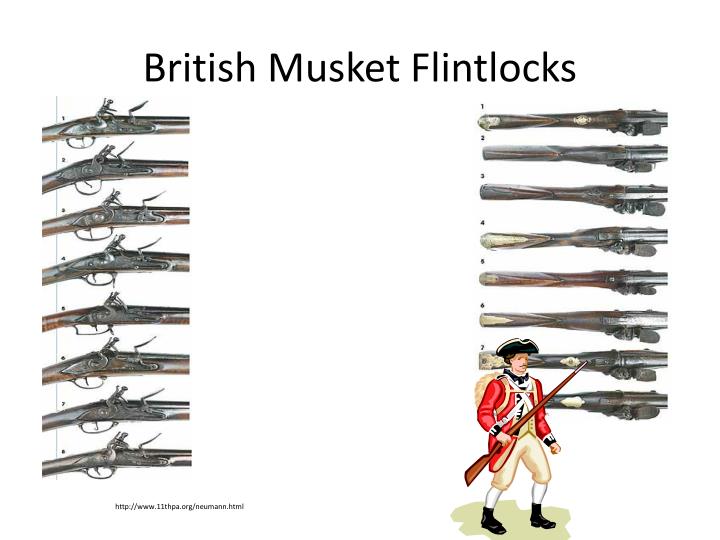The infographic, titled "British Musket Flintlocks" in black text atop a white background, meticulously displays intricate sections of eight British musket flintlock mechanisms. On the left, a vertical column presents these mechanisms from a side view, numbered 1 through 8 from top to bottom. Each model is detailed with ornate designs, primarily in shades of grey, silver, brown, and white. To the right, another column features the same musket mechanisms viewed from the bottom, also numbered 1 through 8, though the eighth is partially obscured by a clipart image of a redcoat soldier. The soldier, from the Revolutionary War era, stands in front, clad in a red coat, tan pants, white socks, black boots, and a black hat, sporting a mustache and brown hair. The image offers a comprehensive comparison of the musket flintlocks' firing mechanisms from different perspectives, emphasizing their historical craftsmanship and utilitarian design.